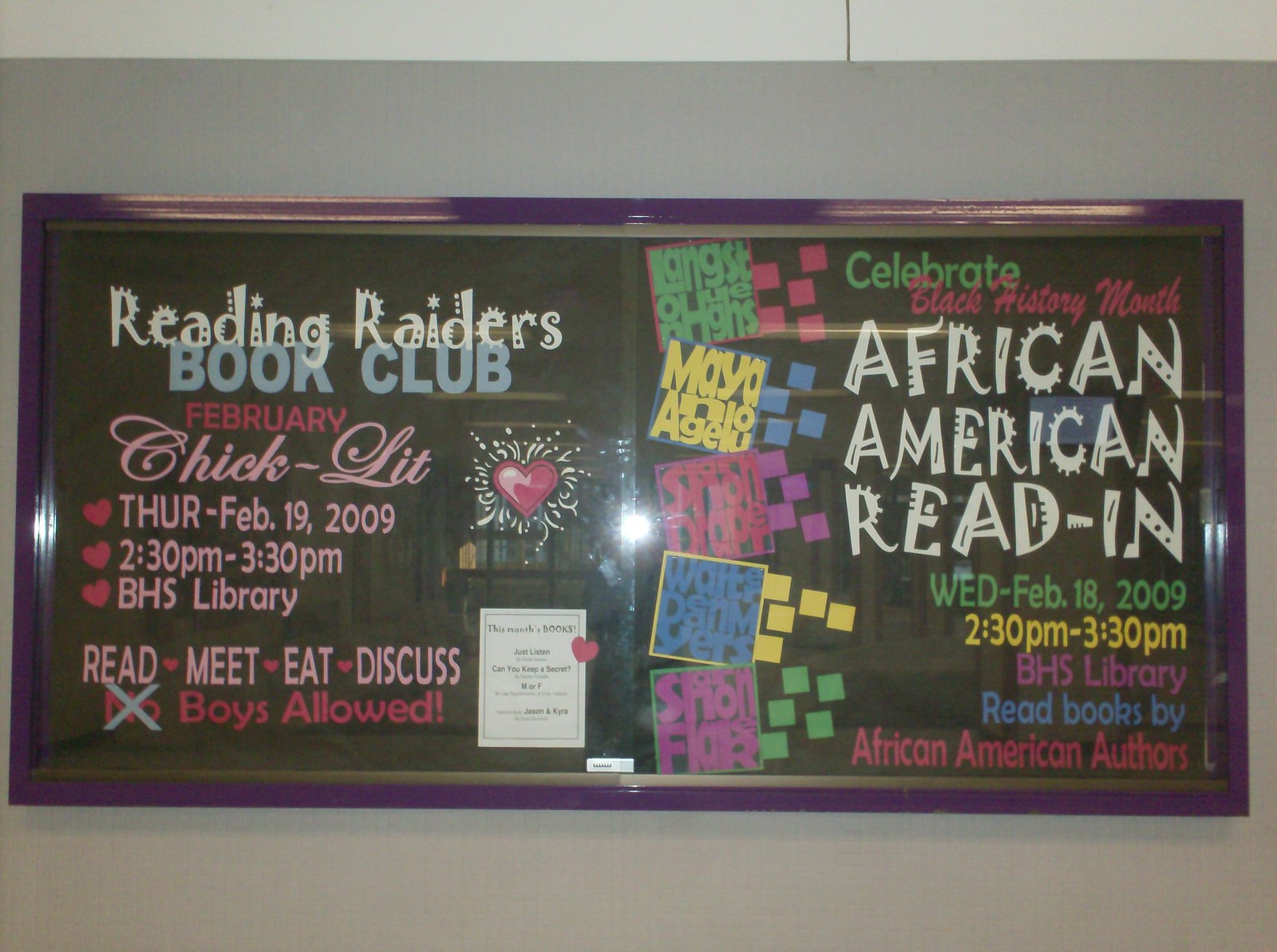This poster, set against a gray wall, features a vivid purple frame that encloses a long rectangular space, wider left to right. It is divided into two sections, with vibrant, colorful lettering against a mostly dark background. The left side promotes the "Reading Raiders Book Club," highlighted in white and light blue text. Underneath, it announces "February Chick-Lit" in eyecatching pink letters, along with three small hearts aligned vertically. Beneath this, details in pink and red include an event on "Thursday, Feb 19, 2009, from 2:30 p.m. to 3:30 p.m." at the "BEHS Library." It encourages participants to "Read, Meet, Eat, Discuss," with an emphatic "No Boys Aloud" marked with an X.

On the right side, the poster celebrates "African American Reading" with green, yellow, blue, and red lettering. This section announces a "Read-in" event for "Wednesday, Feb 18, 2009, from 2:30 p.m. to 3:30 p.m.," also at the "BEHS Library." It encourages attendees to "Read Books" and "Buy African American Authors," with a red heart and radiating white lines adding a festive touch. Both sections of the poster are rich with colors like pink, green, yellow, and red, creating a vibrant and engaging visual centerpiece.